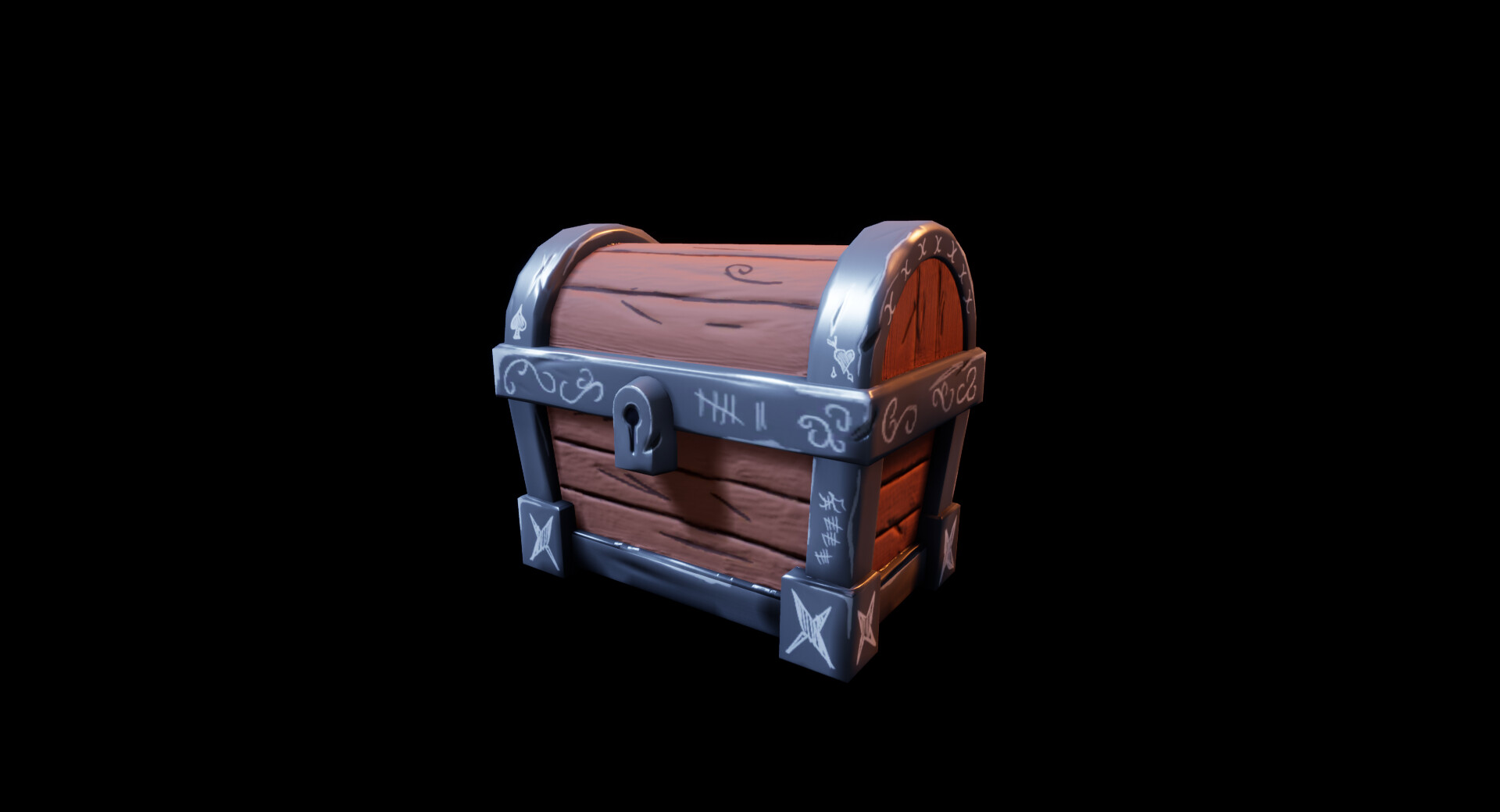The image showcases a digital rendering of a small, brown wooden treasure chest with a curved top, encased in a grayish-silver metallic frame, giving it a toy-like appearance. The chest is centered and tilted slightly to the left against a completely black background, creating the illusion of it floating. Prominently displayed in the center of the chest is a keyhole. The metal parts of the chest are adorned with white chalk lines and scribbles, including random markings and tallies, as well as X's at the bottom corners and a drawing resembling the number 7 near the keyhole. On the far left side, there seems to be an image resembling a spade. Overall, the chest appears to be a child’s toy replica, not an authentic or antique item.